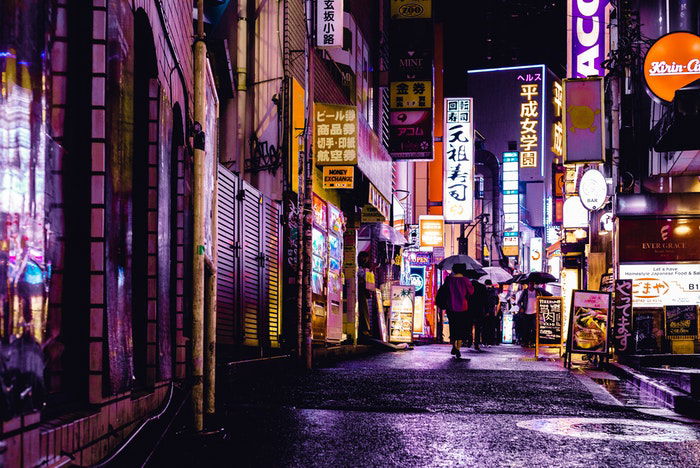The image depicts a vibrant nighttime scene in a bustling urban alleyway in a highly populated part of an Asian city, possibly Tokyo. The atmosphere is dominated by a myriad of neon-lit signs and billboards, all adorned with Japanese kanji characters and a few in English, including a prominent "Kirin" advertisement. The street is flanked by various shops, some of which display images of food items, contributing to the lively ambiance. A trio of people can be seen walking, holding umbrellas, suggesting recent rainfall that has left the ground glistening. The vivid neon lights cast a mesmerizing glow in shades of white, pink, purple, yellow, and blue, creating an almost cyberpunk, futuristic feel.